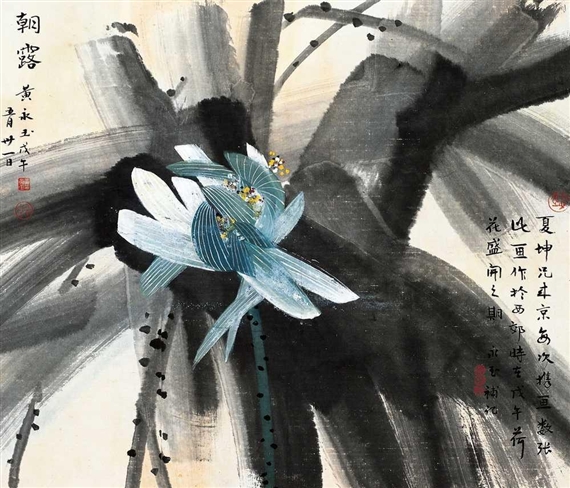The image is predominantly gray and black, with a striking aqua or teal flower that serves as the focal point. The flower, centered slightly to the left, features light blue petals with darker blue centers adorned with intricate white and yellow dots and veins. This vibrant bloom appears to rest atop a series of gray, black, and charcoal lines, resembling branches or vines, adding depth to the white or cream-colored canvas. The upper left corner of the image contains two vertical columns of black Asian characters, while the middle bottom right corner features three additional vertical columns. Scattered throughout the image are a few red characters, notably near the upper middle right and lower bottom right areas.